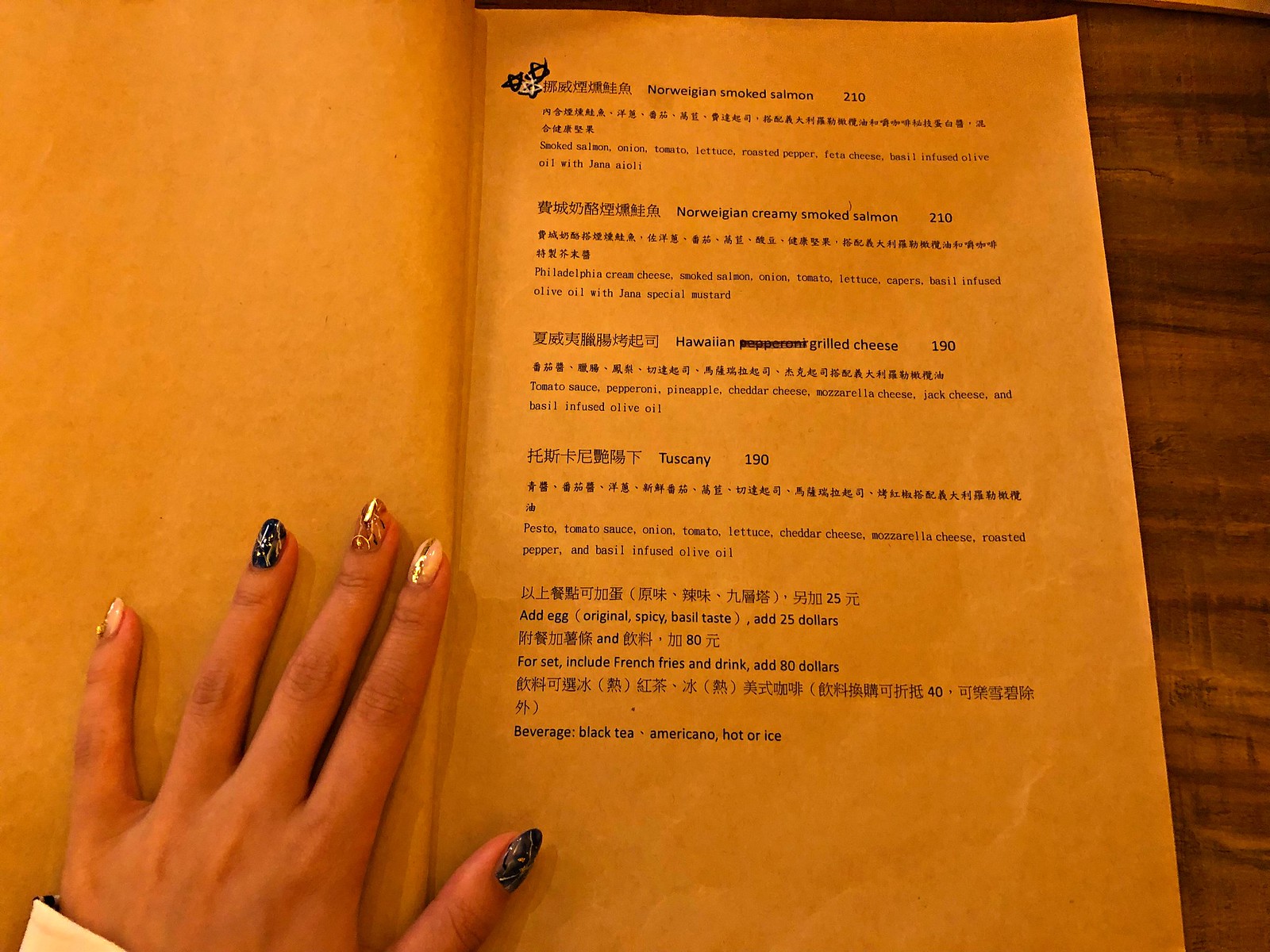This photograph features a tall, narrow rectangular restaurant menu, likely from an establishment in Asia, given the presence of Asian characters on the menu. The menu is text-only, with no images, and provides English translations beneath the Asian script. This particular page of the menu lists five different options. Positioned on a brown wooden table, the menu is being held open by a woman's hand visible on the left side of the image. Her long, likely artificial fingernails are each uniquely painted with intricate designs in shades of gold, white, and brown or black.